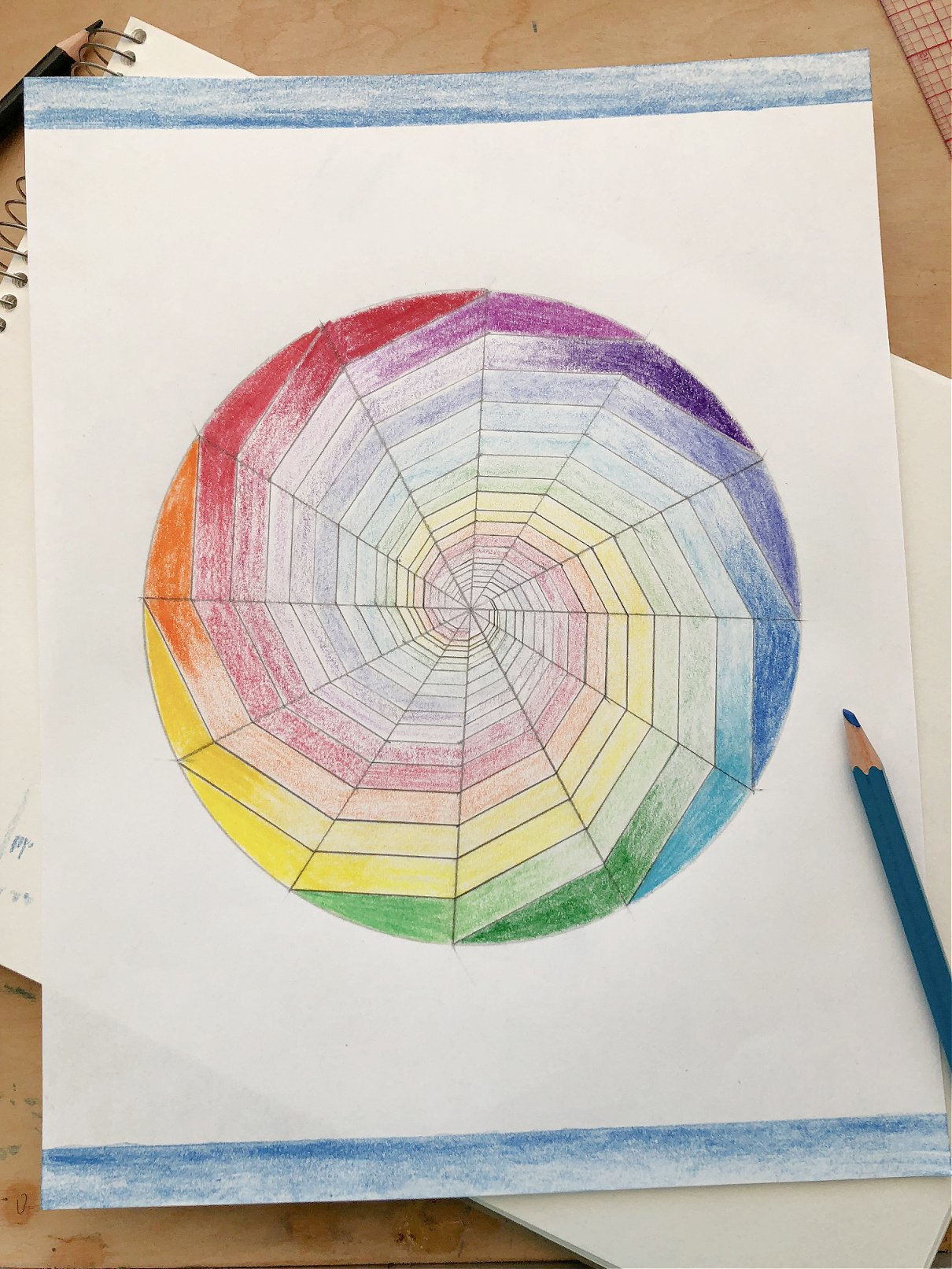The image is a detailed and colorful drawing done on a white piece of paper, depicting a circular symmetrical pattern that resembles a spiderweb. The intricate design features lines radiating symmetrically from the outer edge towards the center, creating a swirling motion that enlarges with each loop. Surrounding the web-like structure are vibrant hues of yellow, green, blue, purple, and red, which progressively fade into lighter shades—such as pink for red, light orange for orange, and lavender for purple—as they move inward toward the center.

The drawing is framed by a horizontal blue strip at both the top and bottom of the paper, inside of which is a subtle hint of white, suggesting it was partially filled in with colored pencil. On the right side of the paper lies a blue pencil, recognizable by its blue tip and a brown segment between the paint and the tip. Additionally, there is another pencil visible in the top corner of the page. The artwork rests on an artist’s pad of paper, which in turn lies on a brown table, adding a tactile element to the composition.